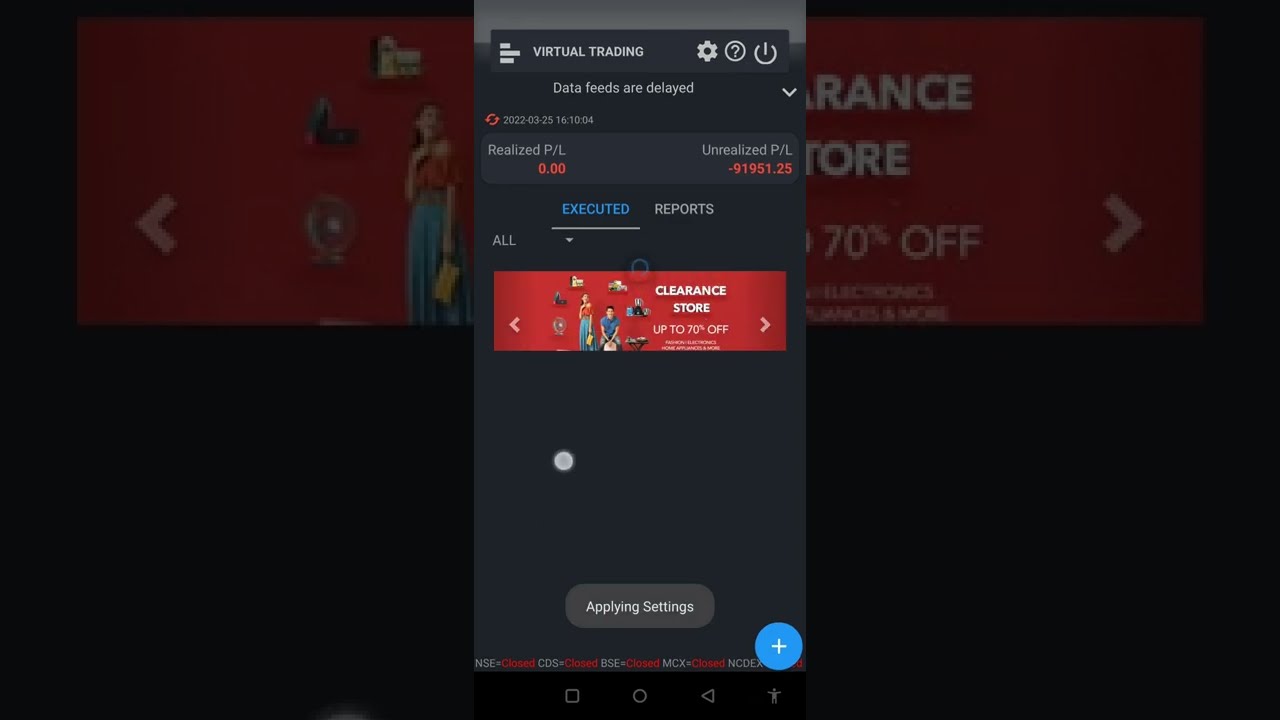The image depicts a mobile screenshot of a trading app focused on stock trading. The app prominently displays "Virtual Trading" at the top, along with a gear icon, a question mark, and a power button. Below this, the app shows financial details: "Realized P/L" at $0.00 and "Unrealized P/L" with a significant unrealized loss of $91,951.25 in red text. Further down, it indicates that a trade has been executed, with sections labeled "Executed" and "Reports." Along the bottom is a banner ad for a clearance store offering up to 70% off, featuring images of a woman, a fan, and several products. The background is predominantly black, with navigational buttons such as a square, circle, triangle pointing left, and a person icon visible at the bottom.